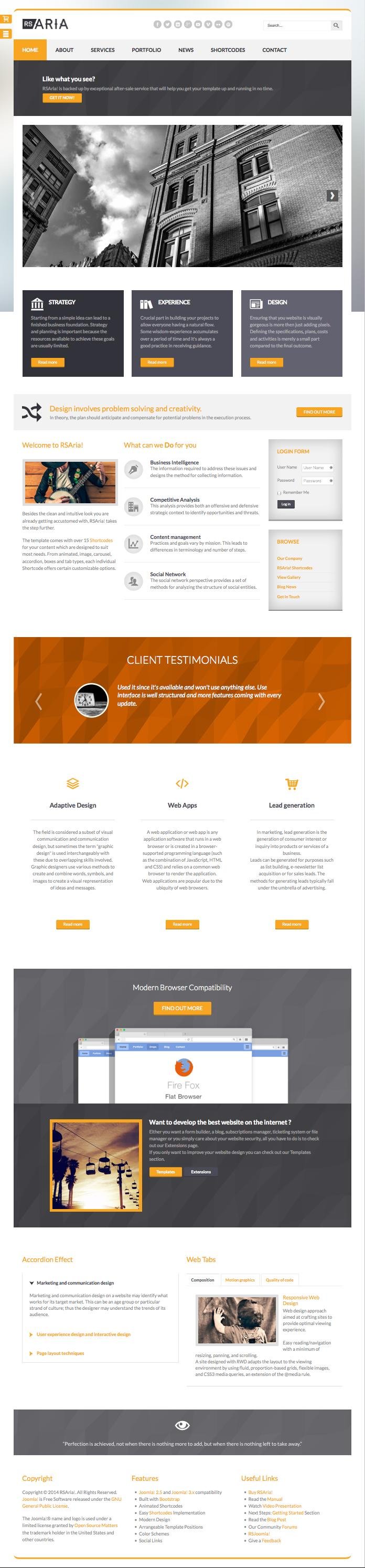This is a detailed screenshot of a smartphone displaying a comprehensive web page for a company named RSARIA. The page features "Area" in bold black letters on the far left, prefixed by "RS" in a small black banner. Centralized in the header, there are several gray social media icons, though they are somewhat blurred and difficult to distinguish clearly. Below these icons, a search bar is prominently placed. 

The navigation menu beneath the search bar includes an orange "Home" button, followed by links to "About," "Services," "Portfolio," "News," "Short Codes," and "Contact." Beneath this, a black banner asks "Like what you see?" above an orange call-to-action button inviting users to "Get it now.”

The main body of the page features a black-and-white image of a tall brick building with elegant, old-fashioned window frames, set against a backdrop of clouds. Below this image are three gray boxes labeled "Strategy," "Experience," and "Design," each with a small icon – a building with columns, three books, and a drafting pencil, respectively. Each box includes an orange call-to-action button.

Further down, a gray banner showcases a pair of intersecting arrows with the phrase "Design involves problem-solving and creativity" in orange letters, accompanied by smaller gray text. Adjacent to this banner is an image of someone playing the guitar, followed by two introductory paragraphs welcoming visitors to RSARIA.

Under these paragraphs is a section titled "What can we do for you?", containing four subsections: Business Intelligence, Competitive Analysis, Content Management, and Social Network, each accompanied by representative icons and brief descriptions. To the right, there are two gray boxes, one featuring a login form and the other labeled "Browse."

An orange banner below highlights "Client Testimonials," next to a small clock icon. The subsequent section is divided into three parts: "Adaptive Design," "Web Apps," and "Lead Generation,” each with explanatory text and an orange call-to-action button.

At the very bottom, a gray section touts "Modern Browser Compatibility" with an "Find out more" call-to-action button in orange. This section is accompanied by an illustration of three computer screens and an image of a ride with cars suspended from a wire.

The footer features an inspirational quote on a gray banner: "Perfection is achieved not when there is nothing more to add, but when there is nothing left to take away," alongside an eye symbol. The footer also includes sections for "Copyright," "Features," and "Useful Links," with these categories in orange and additional text in black beneath them.